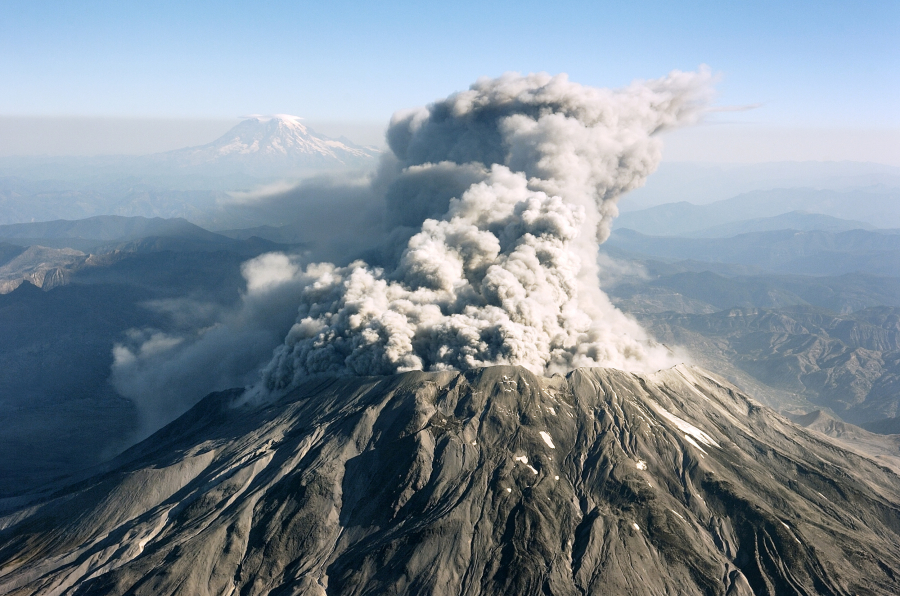The photograph captures a dramatic scene of a volcano in the foreground, actively erupting and spewing a large plume of ash and smoke into the air. The volcano itself is a dark gray and features a flattened, traditional cone shape with a very large opening at the top. The slopes leading up to this opening are gentle, with patches of snow scattered on its surface. A lighter gray ash cloud rises from the volcano, creating a stark contrast against the vivid blue sky that fades into a gradient of darker colors toward the horizon. In the background, distant mountains are enveloped in a haze, enhancing the perception of depth in the image. Among these mountains is another volcano, identifiable by its flat top and white snow cap, which is not currently active. The overall atmosphere is hazy, with the distant mountains more obscured compared to the clear details of the erupting volcano in the foreground.